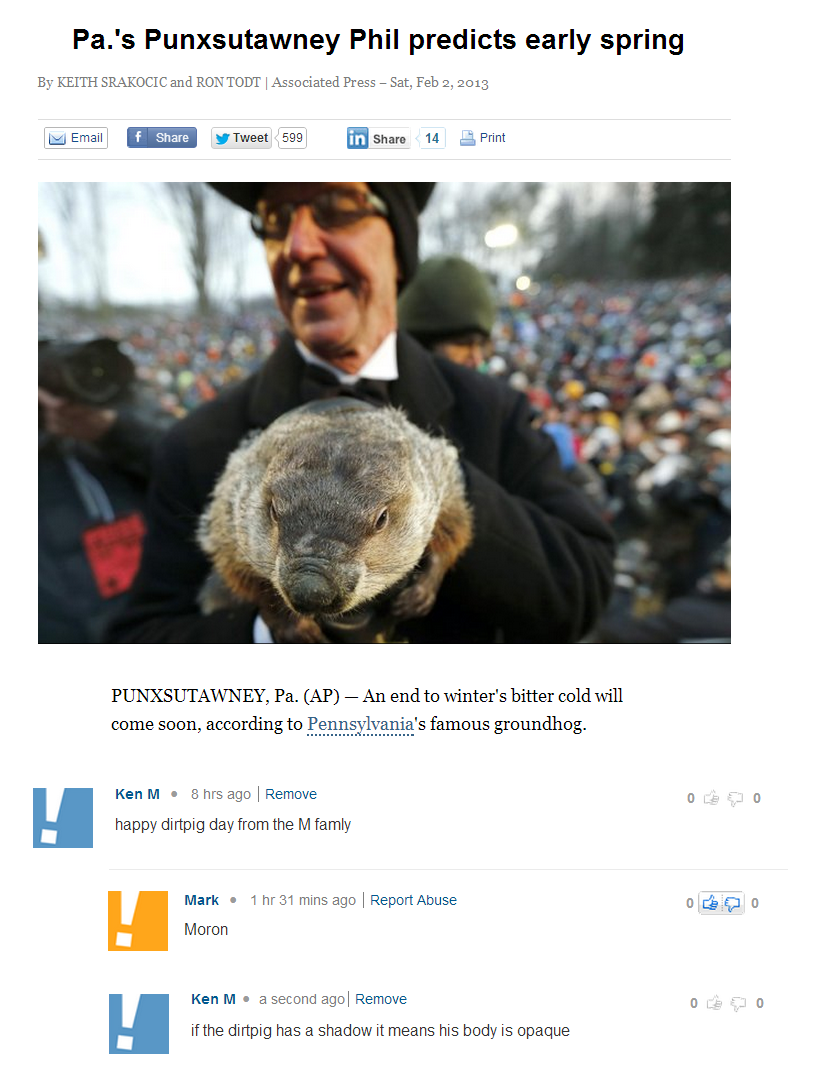**Caption:**

A screenshot of an unfamiliar search page displays an article headlined in bold black font: "Pennsylvania's Punxsutawney Phil Predicts Early Spring." Below the headline, a byline credits two Associated Press reporters and notes the original publication date. A series of share buttons for social media platforms like Facebook and Twitter spans the page’s width, facilitating easy content sharing.

Dominating the page is a large photograph from Pennsylvania's annual Groundhog Day festival. The image features a man in a black suit, hat, and glasses holding Punxsutawney Phil, the celebrated groundhog. Beneath the image, a caption succinctly identifies the groundhog and the event.

Further down, three comments with thumbnail icons are visible; two are blue with a white exclamation point, and one is orange with a white exclamation point. The comments appear to engage in lighthearted banter, adding a layer of casual interaction to the page's content.